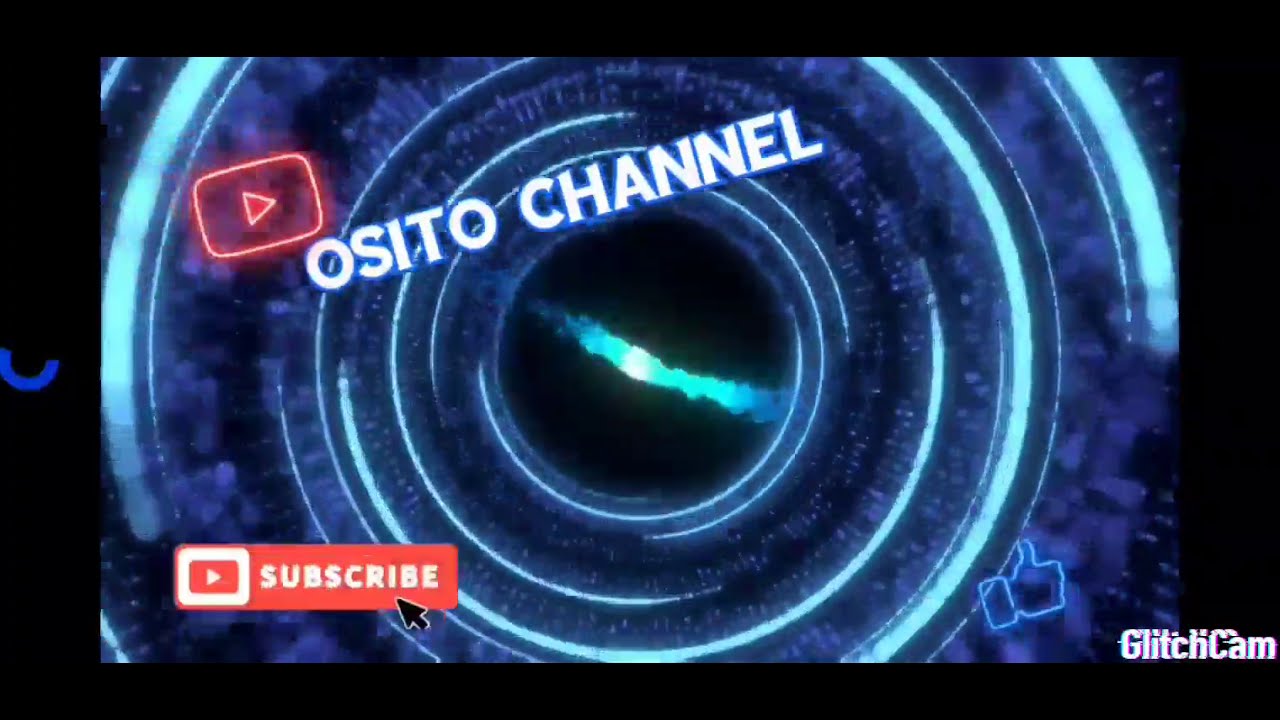This image is a detailed screenshot of a YouTube video promotion. The main focus is a highly zoomed-in image of a camera lens with blue concentric circles that fills the entire frame. There's a diagonal white line cutting across the center of the lens, suggesting light reflecting off the surface.

In the upper left corner, you'll find the YouTube play symbol followed by "OSITO CHANNEL" in bold, white, all-caps letters. On the bottom left corner, there's another YouTube play button next to a red rectangular subscribe button with "subscribe" written in white letters. The bottom right corner prominently features "GLITCH CAM" in white text, just to the left of which is a thumbs-up emoji outlined in blue.

The primary colors of the image include shades of blue, black, light blue, red, white, and gray, giving it a modern, tech-savvy appearance. This structured layout with its bold text and striking visuals suggests a polished promotional banner for a YouTube channel.